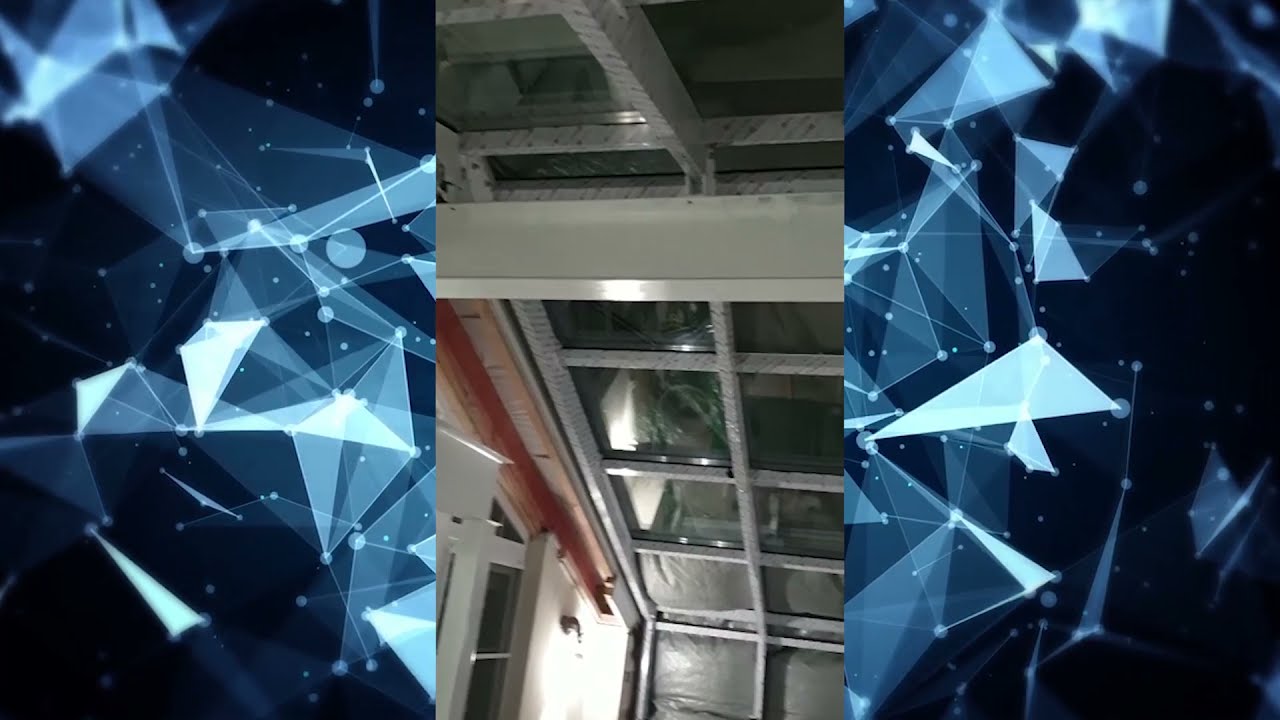In this detailed color photograph, seemingly taken from a cell phone, we observe an interior view of a building, depicted in a portrait orientation and centered against a dark blue background illustration with light blue prisms and circles. The image prominently features a segment of a wall that angles inward to form part of the ceiling, with a continuous window spanning two panes wide embedded into the slant. These windows, framed and divided by horizontal and vertical steel columns, evoke the appearance of partially opened garage doors due to their geometric design and metal structure. The picture is tightly zoomed, giving a close-up view of this architectural detail. Additional elements include a horizontal white beam crossing the top center of the ceiling and, in the bottom left corner, an open white door leading into another room, accompanied by a sconce light fixture to the right of the door and light wood trim above it. The rich colors in the photo include shades of black, light blue, white, gray, orange, and silver, enhancing the image's realistic and representational style.